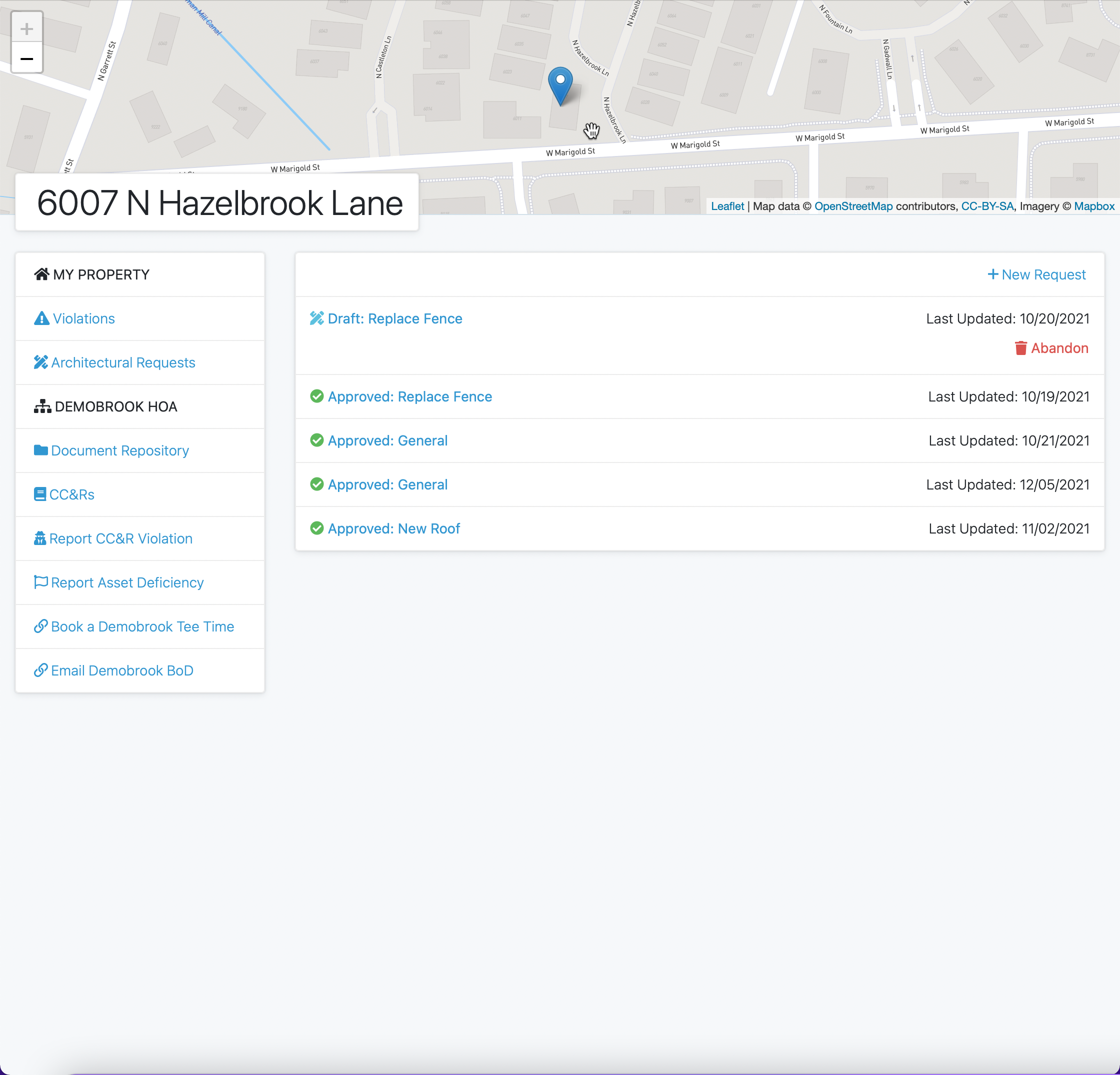A detailed caption for the image could be:

---

This screenshot depicts a location or navigation app interface. At the top of the screen, a map is prominently displayed, featuring a blue and white navigation pin marking an address. The address, visible on the left side of the screen, is listed as "6007 North Hazelbrook Lane." Adjacent to the address, in a smaller font, are references to "Leaflet," "Map data," "OpenStreetMap," contributors, and a registered trademark notice. Below the map and address, a menu labeled "My Property" is shown in bold black font, followed by several submenu items including "Violations," "Architectural Requests," "Demobrook HOA," "Document Repository," "CC&Rs," "Report CC&R Violation," "Report Asset Deficiency," "Book a Demobrook Tea Time," and "Email Demobrook BOD." To the right of this main menu, another section lists various maintenance requests along with their approval status.

---